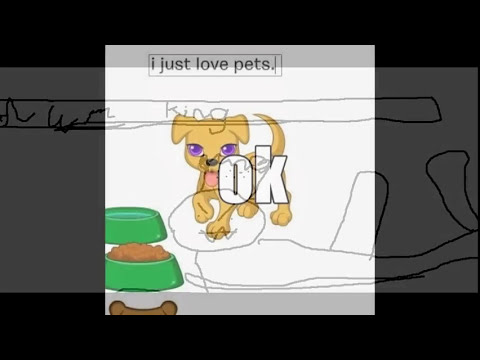This image features a detailed digital illustration of a small tan dog with distinctive purple eyes, set against a vertically rectangular, black-striped background. The composition, reminiscent of an elementary school kid's workbook page, includes a hand-drawn frowny face overlay, contrasting sharply with the more refined drawing of the dog. Above the dog, a printed caption reads "I just love pets." Below this, in a large font with white letters and a black outline, is the word "OK." The dog's name, "King," is inscribed in a child's messy handwriting, and the dog is positioned between two green bowls—one filled with brown kibble and the other empty. Additionally, a brown object resembling a bone is beneath one of the bowls. The overall appearance gives the impression of layers, with some elements looking transparent and others like clip art, creating a whimsical, multi-dimensional effect.